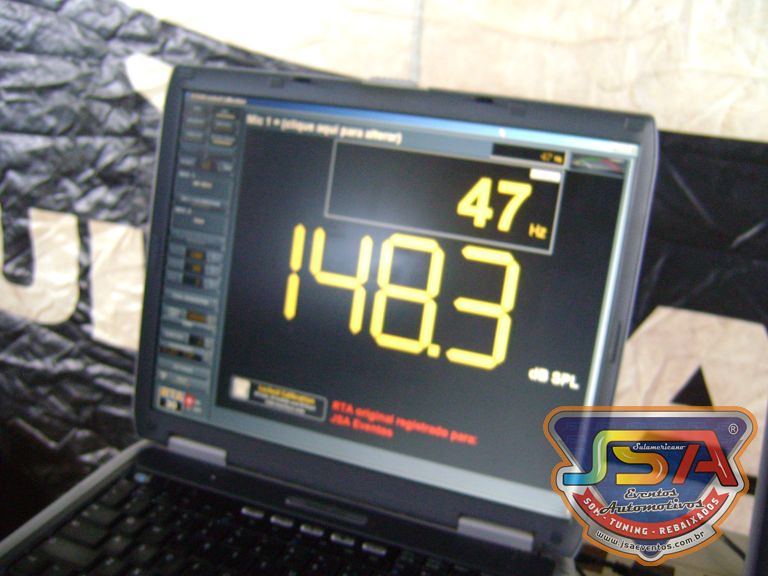Captured in a well-lit room, this image prominently features a sleek laptop positioned centrally on a clean, minimalistic desk. The laptop's screen displays the website URL www.jsaeventos.com.br, indicating it might be showcasing a specific event or content related to the site. The setting suggests a professional environment, perfect for productivity or online meetings. The overall composition of the image underscores the importance of the digital interface in modern workspaces.